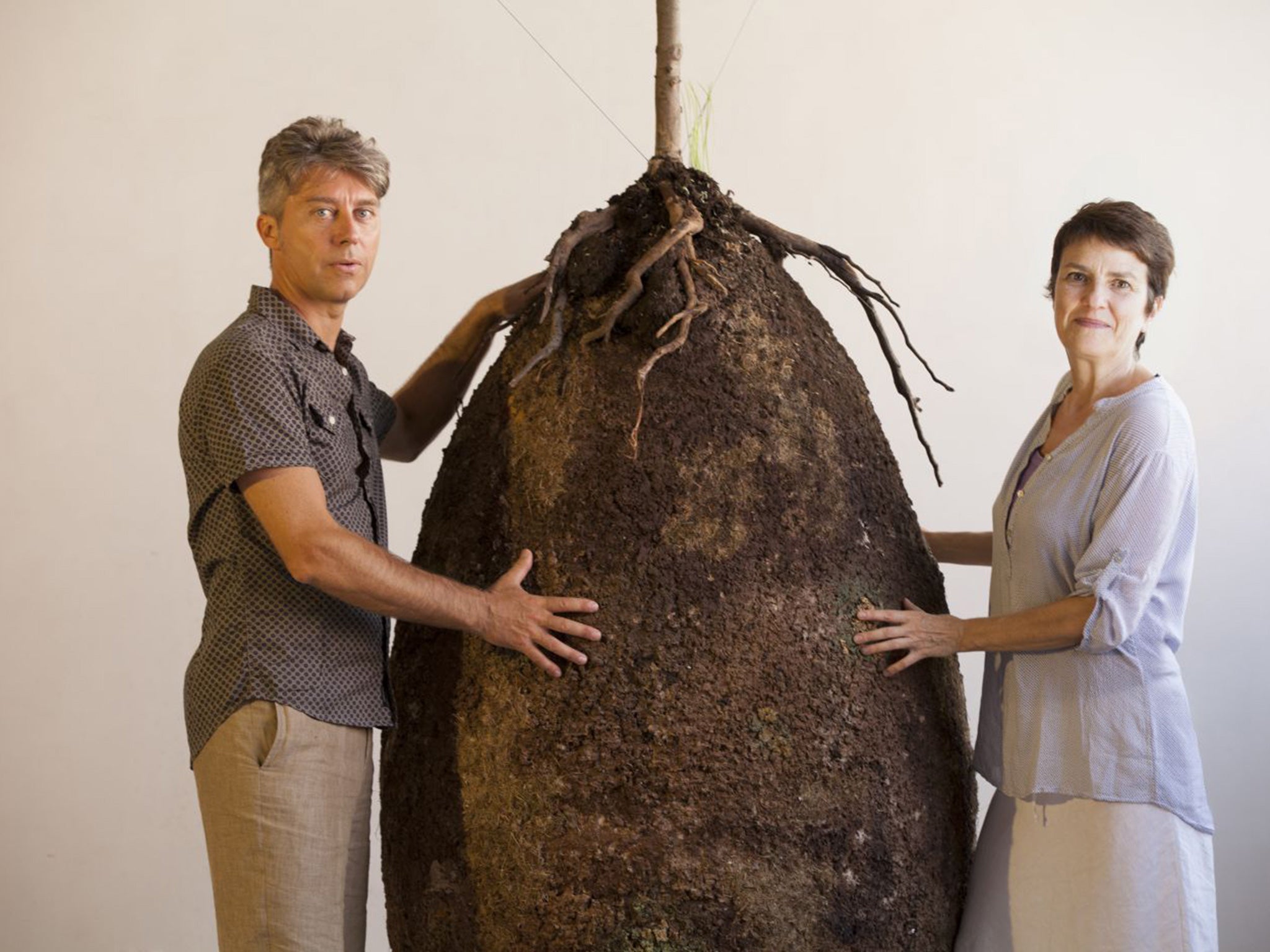In this color photograph, a man and a woman stand on either side of a large, egg-shaped, earthy-looking pod, which is as tall as they are. The pod has a root structure on its top, with the base of a small tree or bush extending out of the frame. Both individuals have one hand resting on the pod, the man's right hand and the woman's left hand, while facing the camera. The background is a beige color, providing a neutral backdrop to highlight the subjects and the pod.

The man, who appears to be slightly above middle age with gray hair, is dressed in a short-sleeve, brown button-up shirt with a striped design, and khaki pants. His mouth is slightly parted. The woman, a brunette with a very short haircut, is wearing a light blue capri top and a white skirt. She is smiling with her mouth closed. This scene evokes imagery of eco-friendly burial practices, where deceased individuals are turned into biodegradable pods to be planted and nourish new life, though the pod here is conspicuously larger than the individuals.